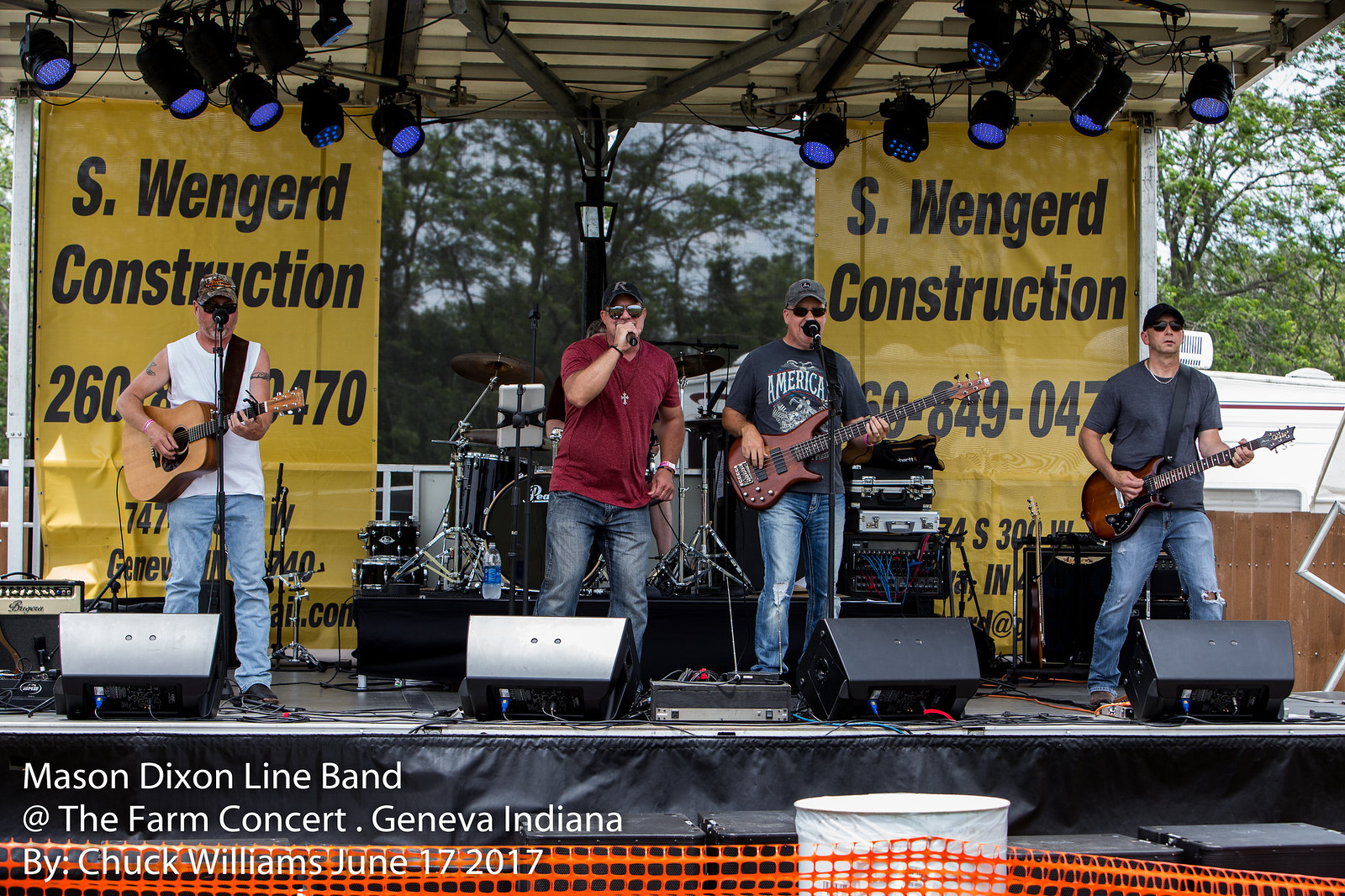The image depicts an outdoor concert taking place on a metal-framed stage adorned with spotlights, lights hanging from the roof, and set against a backdrop of trees. Four Caucasian men are performing, with three playing guitars and one serving as the lead vocalist. The lead vocalist stands at the center, wearing a maroon t-shirt, blue jeans, sunglasses, a black cap, and a cross necklace. He holds a microphone in his right hand and appears to be singing. To his immediate right, a guitarist sporting a green shirt with "America" on it, blue jeans, a baseball cap, and dark glasses stands at a microphone. Further to the right is another guitarist in a gray t-shirt, jeans, sunglasses, and a baseball cap. The man on the left end of the stage wears a white sleeveless shirt and blue jeans, and he is playing a traditional light beige guitar. Both men on the right are playing dark brown electric guitars.

In front of them, there are four large speakers. Behind the band, two identical banners for "S. Wengerd Construction" display the phone number 260-849-0470, although part of one banner is obscured by a performer. A drum set is visible between the two central members, but the drummer is not seen. At the bottom of the image, the caption reads "Mason Dixon Line Band at FarmConcert, Geneva, Indiana by Chuck Williams, June 17, 2017."